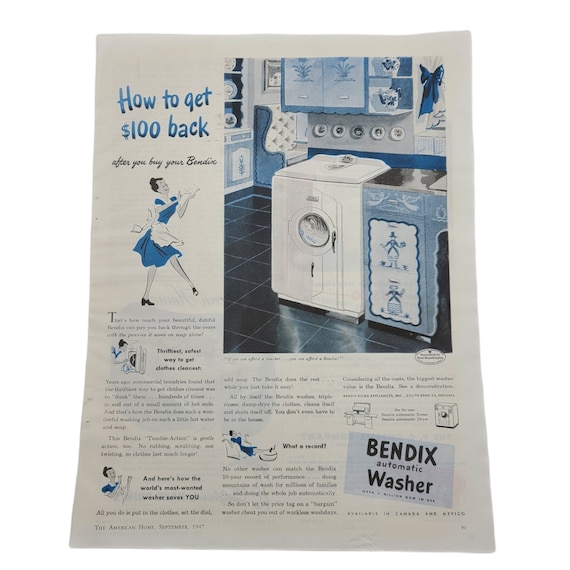This is a detailed picture of an older advertisement, likely from the late 1950s or early 1960s, promoting Bendix automatic washing machines. The vertically aligned rectangular image, probably from a magazine or an instruction manual, features an off-white sheet of paper with visible bends and traces of aging. Dominating the upper left corner, it reads "How to get $100 back after you buy your Bendix," emphasized in larger text, accompanied by smaller, less readable text and illustrative graphics.

Central to the advertisement is a selectively colored illustration, primarily in blue, black, and white, depicting a pristine white washing machine situated in a kitchen or laundry room. The setting is detailed with dark brown square tiles with gray grout on the floor, cabinets overhead, and a window adorned with a curtain tied with a blue bow. Next to the machine, a caricature of a woman dressed in a blue dress with a white apron stands prominently, reinforcing the 1950s domestic theme.

Towards the lower right, the text "Bendix Automatic Washer" is displayed within a small box, reaffirming the product being advertised. The entire composition of the ad, including its hand-drawn elements and vintage aesthetic, captures a nostalgic glimpse into mid-20th century home appliances and their marketing strategies.